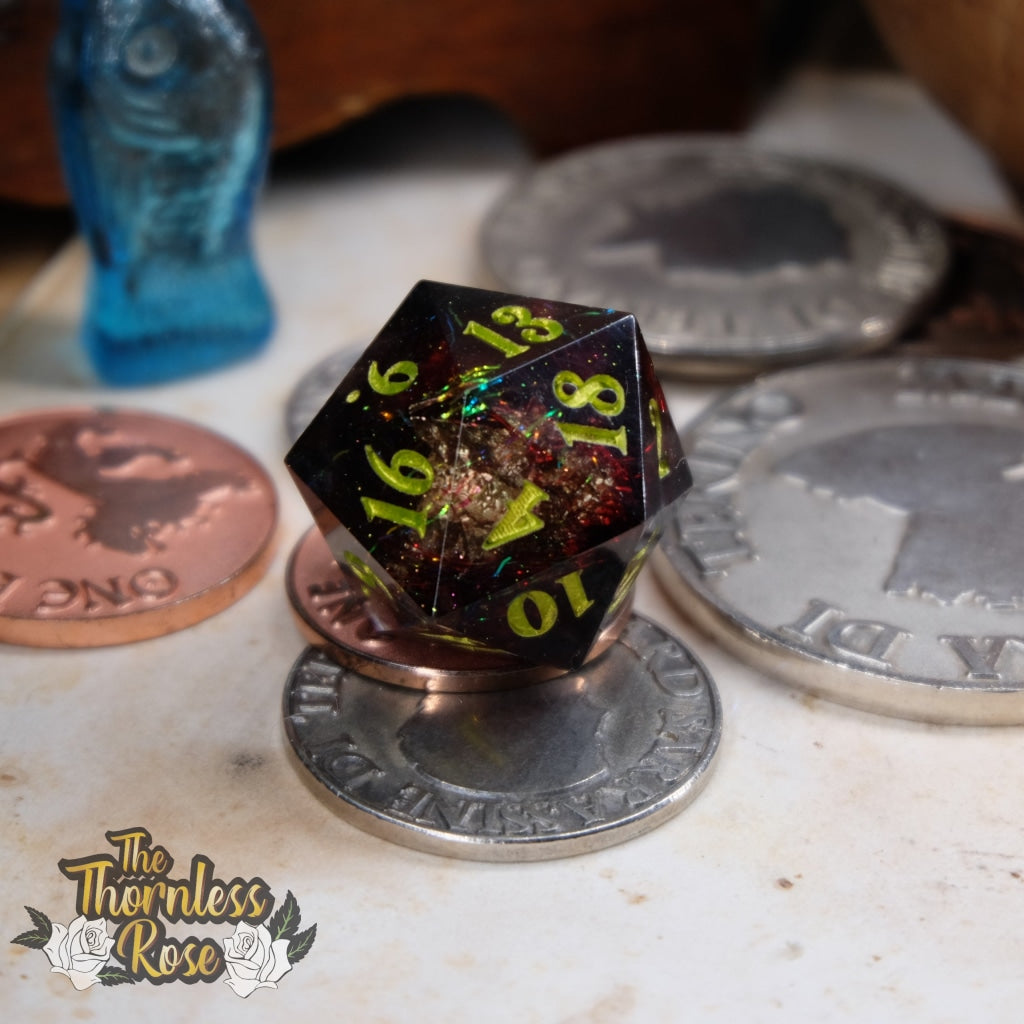This macro photograph captures an intricate scene featuring a transparent black, 20-sided die adorned with rainbow glitter inside, creating a galaxy-like burst. The numbers on the die are painted gold, with visible figures like 16, 9, 13, 18, 4, and 10. The die is perched on a pile of coins, which include both larger silver and smaller copper ones, with the arrangement suggesting a game-like scenario. The coins and die rest on a pale surface, possibly a piece of board, while a blue cup appears in the top left corner of the image, adding a subtle background detail. The bottom left corner of the photo features a watermark that says "The Thornless Rose," outlined in black with white roses, marking the photograph.